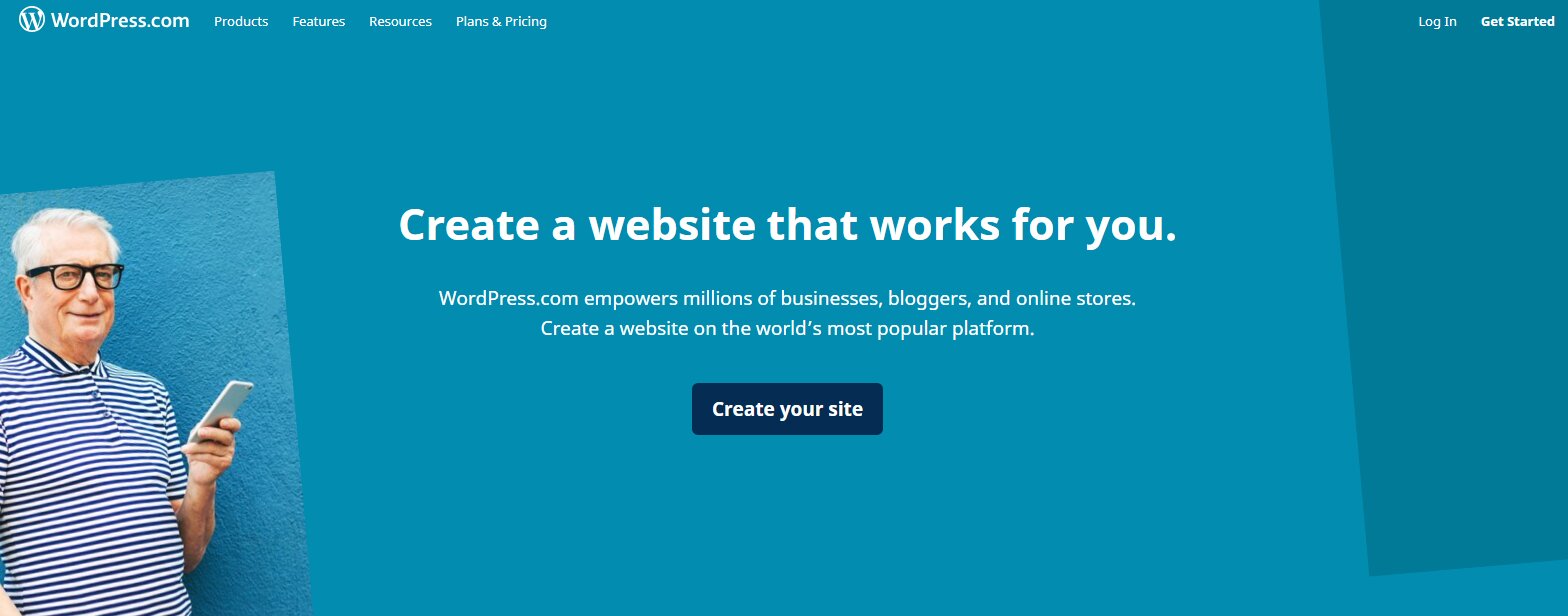**Caption:**

This screenshot showcases the homepage of the WordPress website, predominantly featuring a blue theme. In the upper left corner, the iconic white "W" logo encircled against the blue backdrop signifies the WordPress.com brand. To the right of the logo, a series of navigation buttons labeled "Products," "Features," "Resources," and "Plans & Pricing" facilitate easy site exploration. On the far right of the header, white links for "Log In" and "Get Started" are prominently displayed for user access.

The center of the page presents a bold statement in large white text: "Create a website that works for you," encapsulating the site's core message. Beneath this, further emphasizing the platform's versatility and popularity, is an encouraging line: "WordPress.com empowers millions of businesses, bloggers, and online stores. Create a website on the world's most popular platform." Following this invitation is a prominent dark blue button that reads "Create your site" in white text, prompting users to take action.

Lastly, to the bottom left, an image features an older man with white hair and thick black glasses, donning a striped polo shirt. He is holding a white phone, adding a personal, relatable touch to the professional website atmosphere.